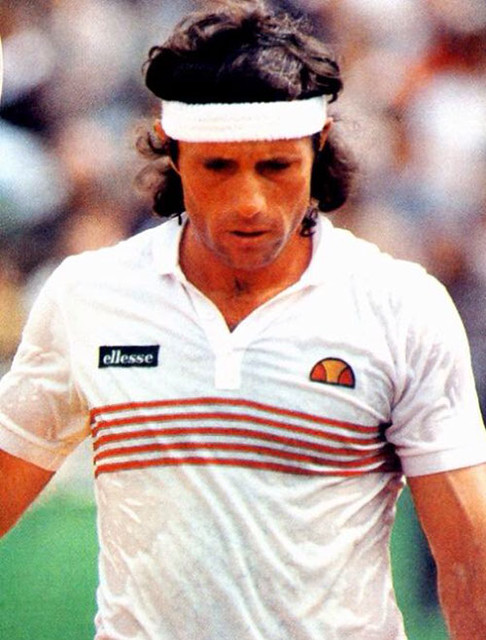The photograph showcases a man with wavy, shoulder-length, dark hair, appearing to be an athlete, possibly a tennis player from the 70s or 80s. He is wearing a white headband around his head and a clean-shaven face. The man, drenched in sweat, giving his white short-sleeve polo shirt a wet, wrinkled appearance, is captured from his head down to his torso. The polo features five red horizontal stripes across the chest, a black rectangle with the letters "ELLESSE" on the right, and an orange and red semicircular logo resembling a tennis ball on the left. The background is highly out of focus, providing a blurred backdrop with indistinguishable elements, hinting at the presence of people. The ground beneath him is green, possibly a grass court, further suggesting a sporting event. The overall vintage quality of the photograph, or perhaps a posterized effect, contributes to its nostalgic feel.